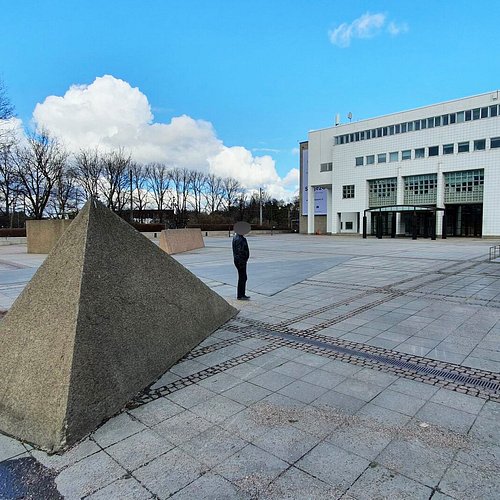The image showcases a detailed and nuanced scene of a large plaza with various geometric stone sculptures, including a prominent triangular-shaped stone in the foreground. At the center stands a man dressed entirely in black, his head noticeably blurred out or grayed over. He faces a substantial three-story, beige-colored building situated directly in front of him. The building's facade features three large garage doors on the bottom level, and rows of small square windows on the stories above. To the left of this building, bare trees stretch up towards a clear, blue sky adorned with puffy white clouds. The plaza itself is composed of worn, square concrete tiles, creating a weathered and aged appearance. Scattered around the plaza are additional geometric stone shapes, adding an abstract element to the scene. The overall setting suggests an autumn day, with the leafless trees and clear skies contributing to a crisp, serene atmosphere.